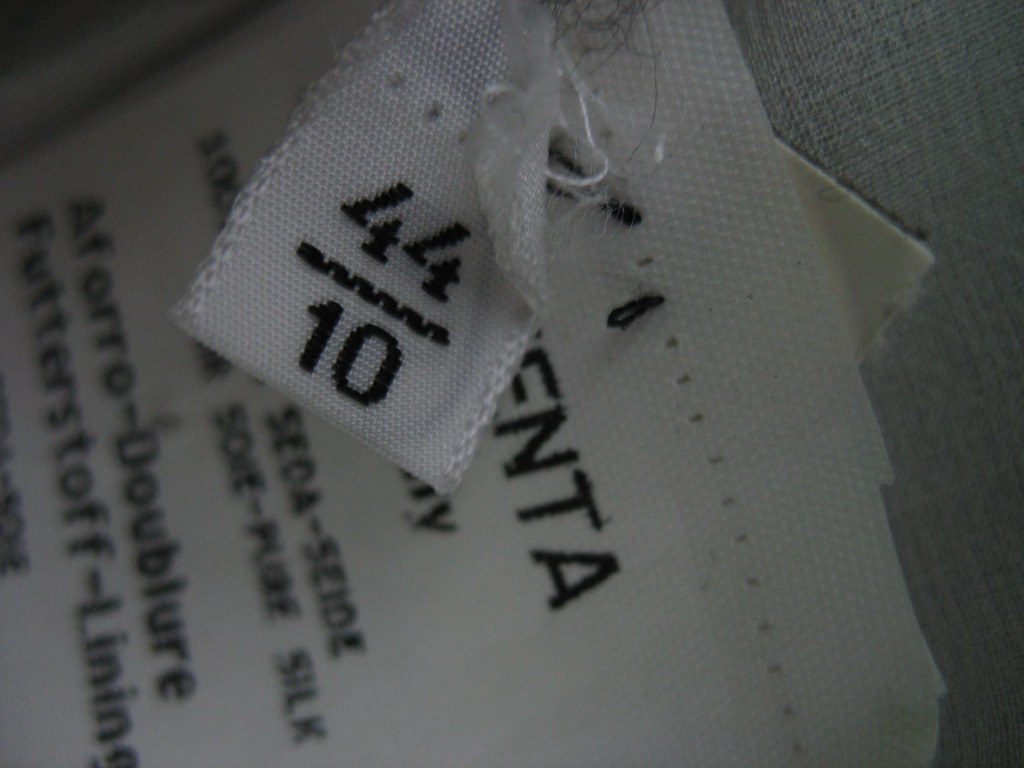A close-up image captures the white fabric tags typically found on clothing, sewn into gray t-shirt material. The photograph highlights two tags placed sideways, making them somewhat difficult to read. The smaller tag in the foreground features black text with a prominent '44', followed by a black bar and '10', possibly indicating size measurements. Behind it, a larger tag displays 'ENTA' in bold black font with additional smaller text and numbers below it, though these details are not clearly legible due to the orientation and zoomed-in nature of the photograph.